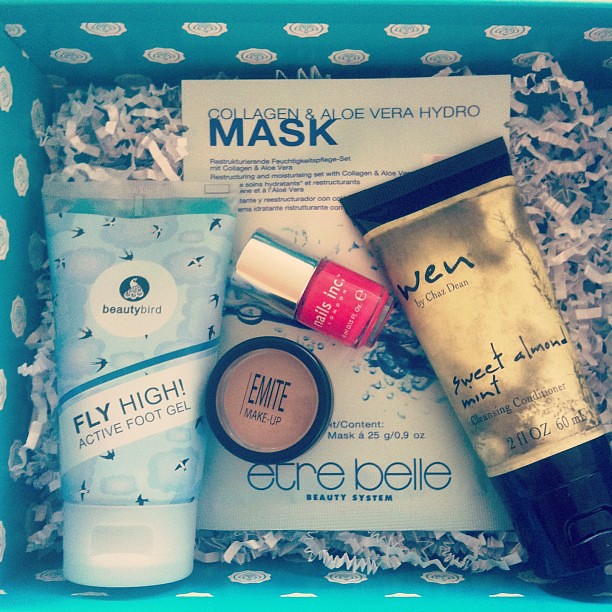The image depicts a meticulously arranged gift box with a blue exterior adorned with white floral patterns resembling polka dots. Inside the box, a bed of crinkled white paper serves as the packaging material for an assortment of beauty products. 

On the left, there's a tube of Beauty Bird Fly High Active Foot Gel, distinguished by its label featuring small black birds and white clouds on a blue background. In the center, a circular plastic container of beige and black Emite Makeup is visible through its clear acrylic lid. Nearby, a Collagen and Aloe Vera Hydro Mask from the brand Etre Bell Beauty System is present, marked as 25 grams or 0.9 ounces. Adjacent to it is a mini bottle of pink nail polish and a Sweet Almond Mint Cleansing Conditioner by WEN, W-E-N, by Chaz Dean, housed in a gold-colored tube with a black cap.

The detailed presentation of the products against the white crinkled paper backdrop inside the embellished blue box suggests a carefully curated selection intended for gifting.